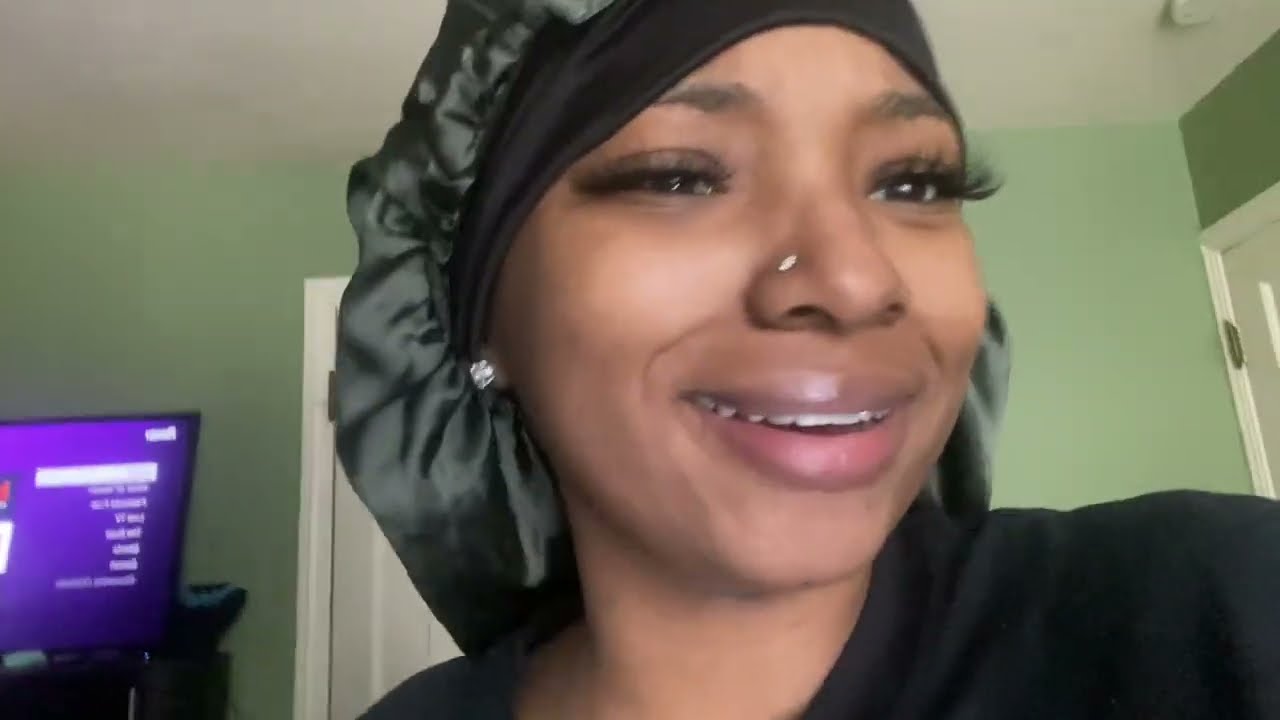A close-up selfie captured with a webcam shows a smiling African-American woman in her 20s or 30s. Her open-mouth smile reveals the bottom of her top teeth. She has smooth skin, long black eyelashes, and sports a nose piercing on the right side. Her ears are adorned with diamond-studded earrings. She's wearing a head covering typically worn for sleep, featuring a black band around her forehead and a fluffy dark green section at the back. Her attire is a simple black t-shirt, visible from the neck up.

The background suggests she’s in a personal space, likely a computer room or living room, characterized by light green walls, a white ceiling, and at least one white door. On the left side of the image, partially visible, is a computer monitor displaying a purple screen with illegible text. The purple screen hints at a Roku device, indicated by the brand name appearing reversed. The setup includes another white door to her left (right side of the image for the viewer), and there might be what resembles a fire extinguisher near the ceiling area, though this detail is not as clear. The overall setup points to an indoor environment, capturing a moment of casual comfort.